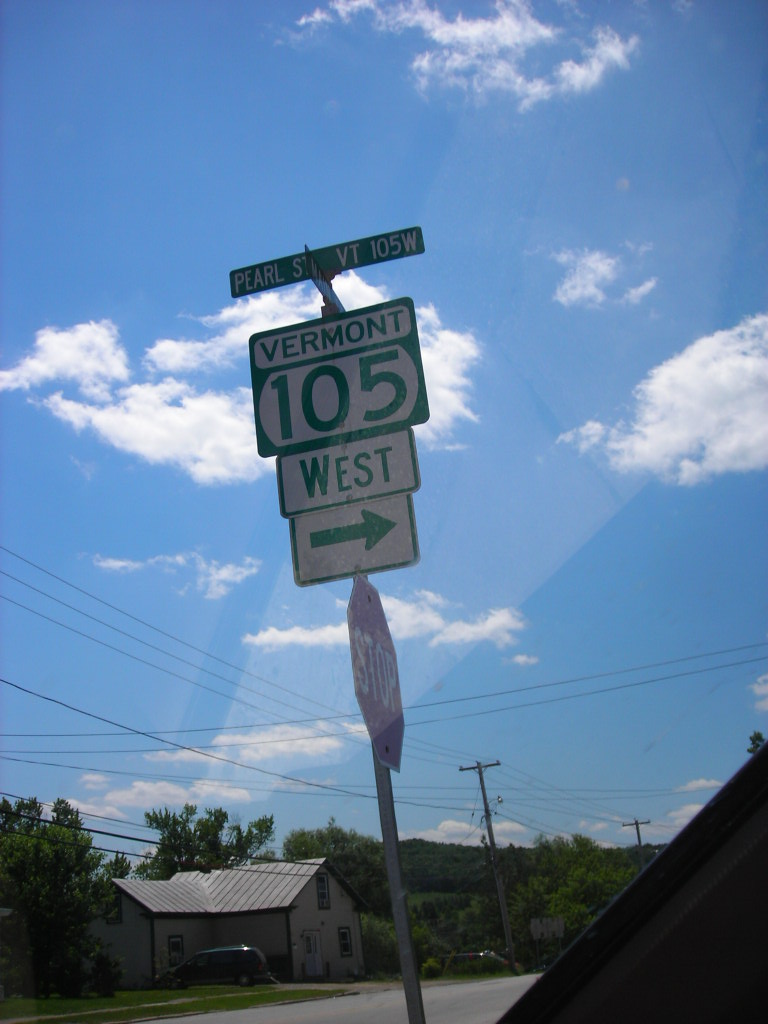This photograph, seemingly taken from inside a vehicle through a window, captures a detailed street scene dominated by a series of street signs in the foreground. The primary sign at the top reads "Pearl ST VT 105 W" in green and is positioned alongside another street sign that is obscured and unreadable. Below, a green box with "Vermont 105" in black text and another white box with "West" followed by a right-pointing arrow are visible. These signs, mounted on a metal pole, are directly above a prominent red stop sign with white lettering, indicating the vehicle is likely halted at this intersection.

In the backdrop, a charming two-level house with a beige facade and a dark brown metal roof is visible on the left side. Parked in its driveway is a large vehicle, possibly an SUV or a van, alongside a well-maintained lawn and sidewalk. Adjacent to this house, a large telephone pole stands among various trees with telephone wires stretching across the upper part of the image. The scene is brightened by a brilliant blue sky dotted with white clouds, adding to the vividness of the street view. The reflection in the window from which the photo is taken subtly reveals the context of the photographer's position inside a vehicle.